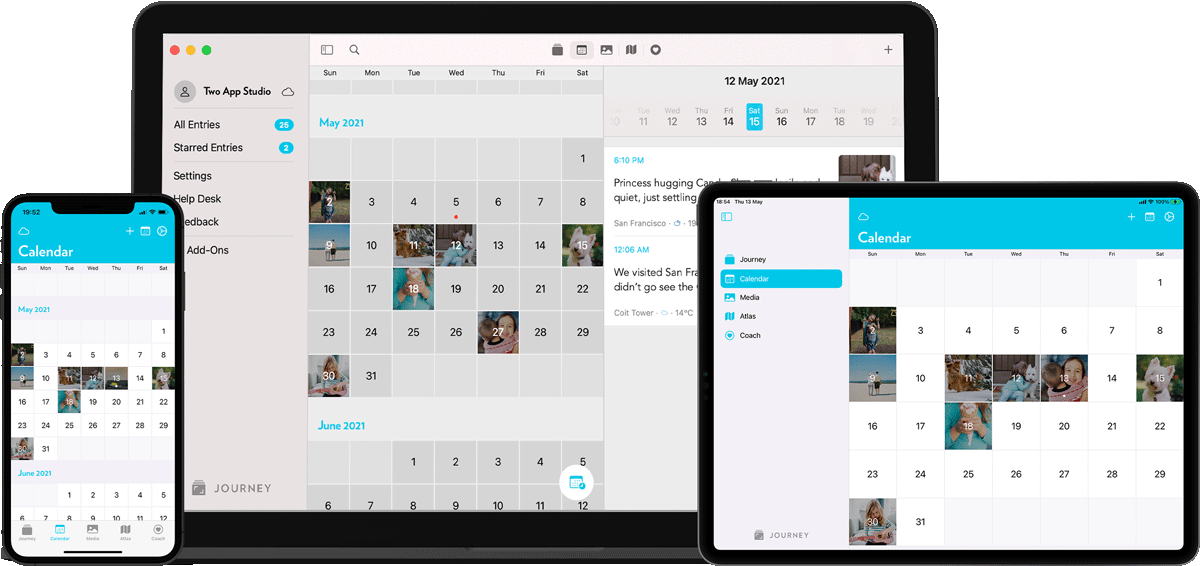"This image showcases a mock-up of a calendar application displayed across multiple devices: a smartphone, tablet, and laptop. On the left, the smartphone, resembling an iPhone, prominently features a calendar app with a blue header reading 'Calendar' and various calendar options below. Each date square includes small photographs, though the specific month is not discernible.

Adjacent to the smartphone, on the right, a tablet mirrors the same calendar interface with the blue header and date squares containing photos. Behind these devices, at the center, an open black laptop displays the calendar application within an Apple interface. The laptop's upper left corner has the distinctive red, yellow, and green window control buttons.

The laptop's calendar view has a mauve background instead of blue and reveals additional options like 'All Entries,' 'Starred Entries,' 'Settings,' 'Helpdesk,' and 'Feedback.' The date squares on the laptop are gray, contrasting with the white squares on the mobile devices, and show more information with visible months noted as May 2021 and June 2021. Overall, this mock-up illustrates the responsive design of the calendar app across these devices."